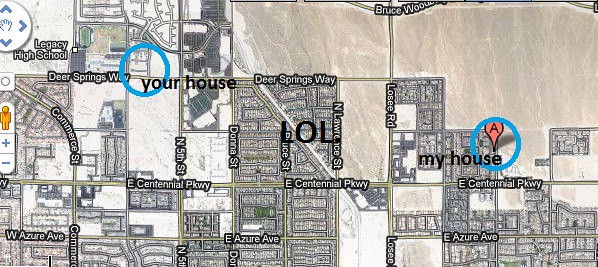The image is a detailed rectangular map segment, presumably from Google Maps, displaying a specific area. Located in the upper left corner of the map are orientation arrows indicating the cardinal directions: north, south, east, and west. A Google Maps-like interface element with a plus and minus sign is visible, allowing for zooming in and out.

The map illustrates several blocks of a neighborhood with two blue circles marked "Your House" and "My House," respectively. In between these two points, at approximately one block distance, there is a label that reads "LOL." Prominent streets such as East Centennial Parkway, Deer Springs Way, and Azure Avenue are clearly marked. 

While the map mainly appears in shades of brown and white, there is a small green area indicating Legacy High School. The overall aesthetic of the map suggests it may have been rendered in a sepia tone or had a brown wash effect applied to certain areas, superimposed on a standard black-and-white Google Maps view.